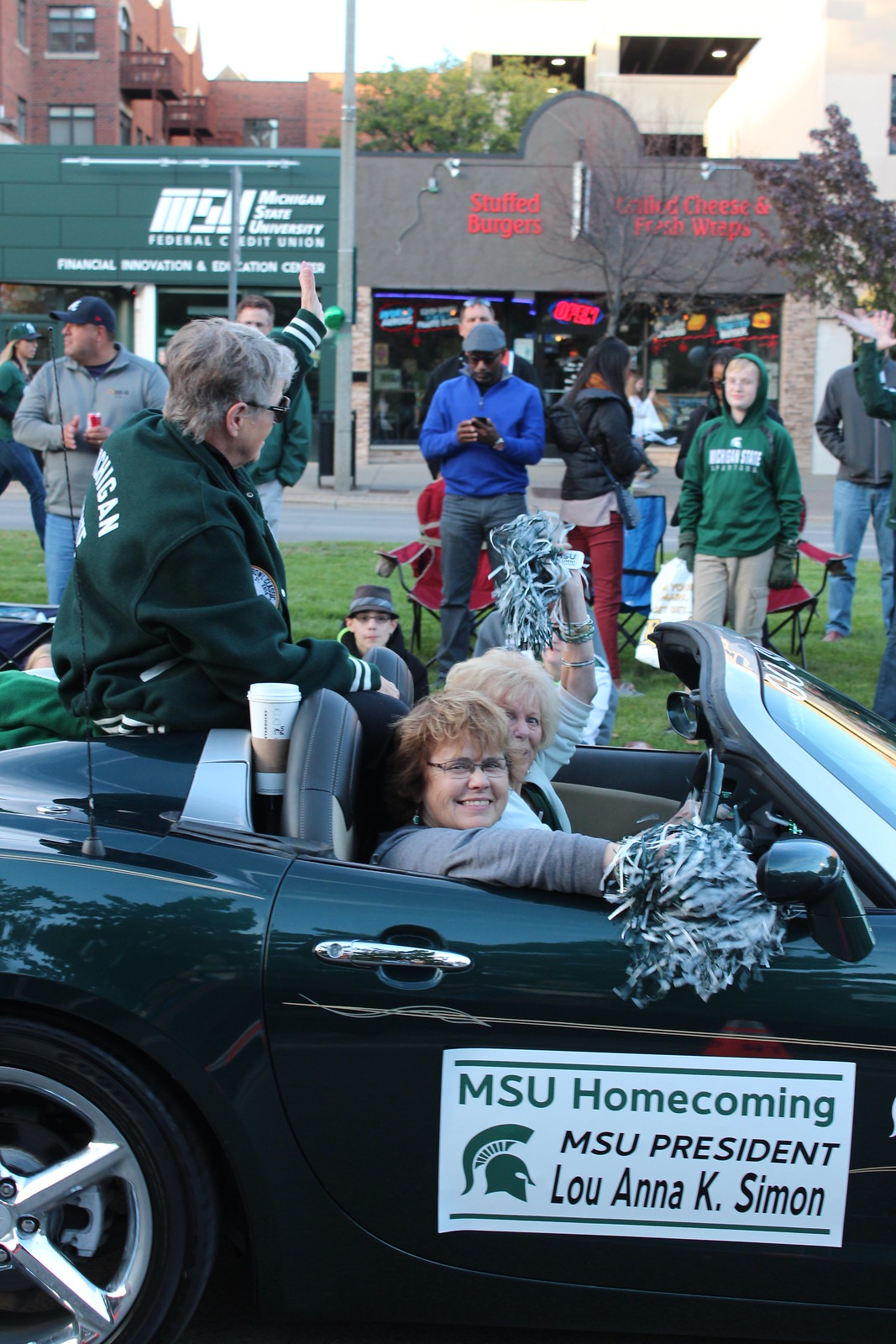In the vibrant scene of an outdoor parade, a dark forest green convertible glides down the street, its roof down to embrace the day. Prominently displayed on the passenger door of the car, a white banner adorned with green lettering reads "MSU Homecoming," accompanied by a Spartan helmet logo and the inscription "MSU President Lou Anna K. Simon." At the front of the two-seater vehicle, two women sit, one with blonde hair at the wheel, and the other with brown hair in the passenger seat, both enthusiastically waving silver pom-poms. An elderly man with gray hair and glasses, clad in a green Letterman jacket emblazoned with "Michigan" on the back, casually perches on the trunk, gazing away from the camera. The scene is set against a lively backdrop, where spectators, some seated in soft collapsible chairs of red and blue, stand along the grass. The surrounding cityscape includes a strip mall with signs for the "MSU Federal Credit Union" and a food outlet advertising "Stuffed Burgers, Grilled Cheese, and Fresh Wraps." This festive moment captures the essence of Spartan pride and community spirit during the homecoming celebration.